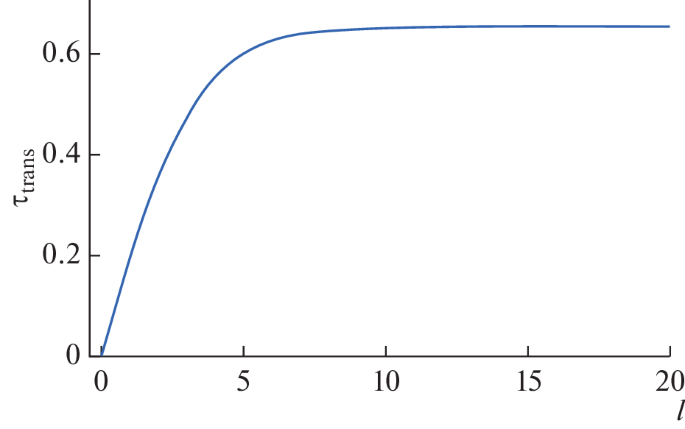The image showcases a detailed graph, characterized by a T-shaped symbol labeled "trans" on the left side. The y-axis of the graph is marked with intervals ranging from 0 to 0.6, progressing through 0.2 and 0.4. The x-axis is labeled with numbers from 0 to 20, segmenting at 5, 10, and 15. At the bottom right corner, there is an L symbol marking the horizontal axis. A prominent blue line begins at the origin point (0, 0) of both axes, rising diagonally until it intersects the x-axis at the 5 mark and the y-axis at the 0.6 mark. Beyond this point, the blue line flattens into a horizontal trajectory, extending up to the 20 mark on the x-axis.